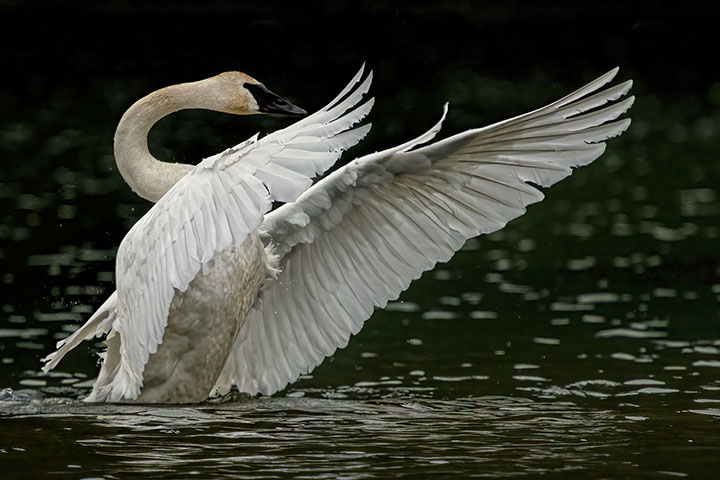This detailed outdoor image captures a white swan gracefully poised on a dark, reflective body of water, possibly a pond or lake, with intricate ripples and some scattered debris visible on the surface. The swan, facing the right side of the frame, is shown in an action shot with its majestic wings spread wide, just skimming the water, suggesting it is on the verge of taking flight or warding off an intruder. Its lower body is submerged, while its elegant, arching neck, reminiscent of the letter 'C', bends forward. The swan features a striking black beak and subtle reddish accents and patterns on its cheeks and neck. The background gradually blurs, creating a bokeh effect that emphasizes the swan's detailed feathers and the overall serene yet dynamic moment.